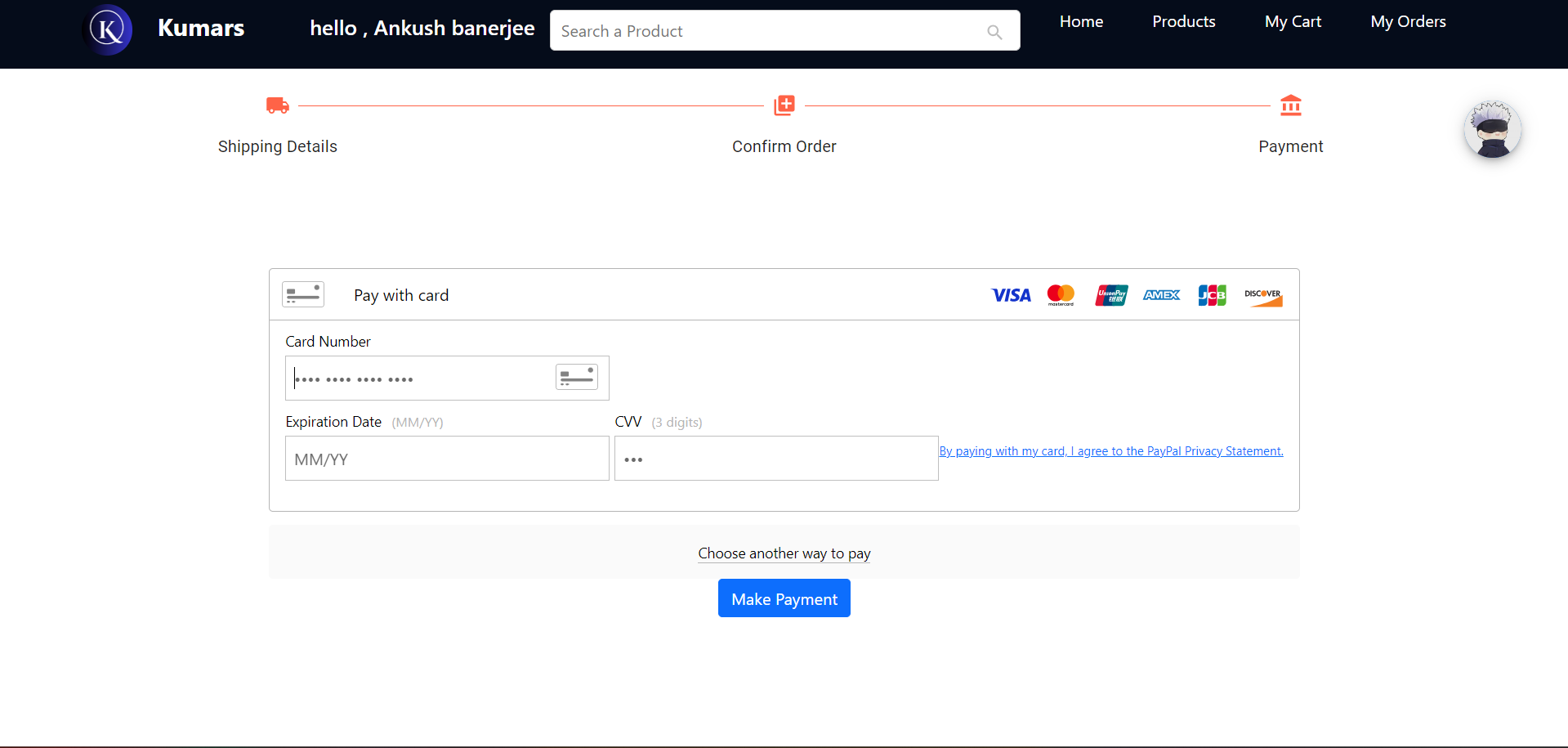This image is a cropped screenshot of a website with a black horizontal header bar occupying around 15% of the total image height. On the upper left of this bar is a white circular logo featuring the letter "K", partially shadowed in medium blue. To the right of the logo, in white text, is the word "Kumars" followed by a greeting "Hello" addressed to Ankush Banerjee. Adjacent to this greeting is a white search bar with the placeholder text "Search a product" in gray, and a magnifying glass icon on the right side. Further right in the header are navigation options labeled in white as "Home," "Products," "My Cart," and "My Orders."

The main body of the website has a white background. Directly below the header is an orange horizontal line spanning the width of the image. To the left of this line is an icon of a moving truck and the label "Shipping Details." Centered along the line is a plus sign within an orange square accompanied by the text "Confirm Order." On the far right of the line is a building icon next to the label "Payment."

Below this horizontal section is a detailed area focused on payment. It includes a segment labeled "Pay with card," displaying various card options to the right with fields to enter card information below. The entire layout suggests a shopping or e-commerce website mid-transaction, specifically during the checkout stage.